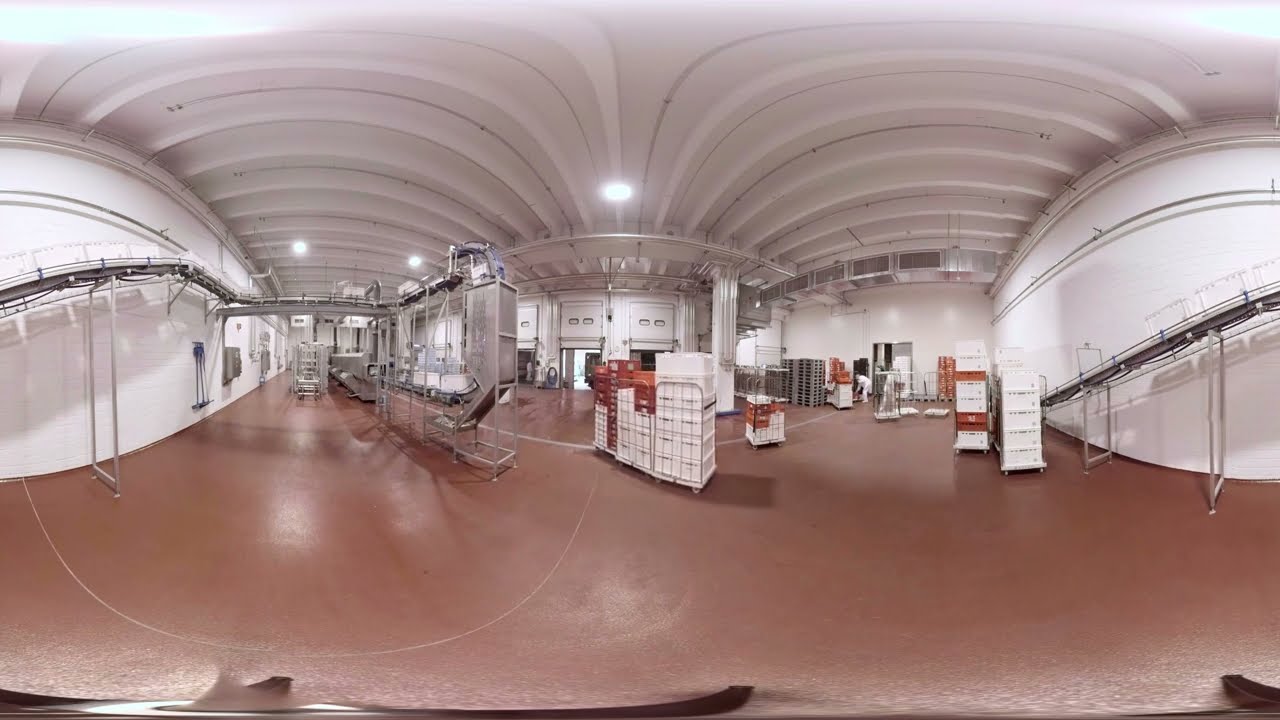The image appears to be an interior shot of a warehouse taken with a fishbowl lens, creating a distinctive curved distortion on both the left and right sides of the picture. This distortion may also suggest the use of a 360-degree camera. The floor is a light reddish or pinkish cement color, which complements the predominantly white walls. The ceiling features a unique M-shaped curve, creating an arch on either side.

On both sides of the image, there are various structural elements, including scaffolding or stairways resembling bridges that connect from left to right. These elements appear almost symmetrical, emphasizing the mirrored effect. There is also a conveyor belt apparatus made of stainless steel on the left side of the image. In the center background, there are three garage doors, likely leading into the structure, flanked by stacks of white and brown boxes, suggesting this area may serve a shipping or storage function.

Additionally, the image includes what seems to be inverted storage bins placed on a rolling dolly, reinforcing the warehouse setting. There is a long steel apparatus visible towards the middle center back, and a possible handrail or track on the left-hand side, which also exhibits a curved or "bubbling" effect due to the camera distortion.